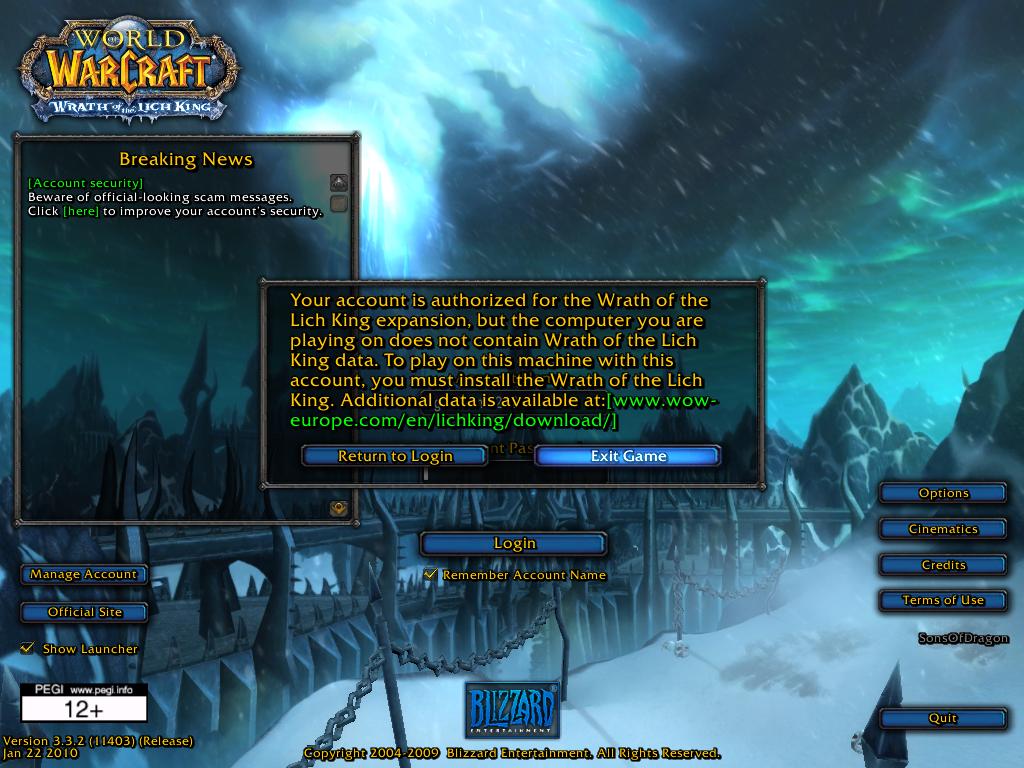The screenshot depicts the login screen of "World of Warcraft: Wrath of the Lich King" captured on a Windows computer. Prominently displayed in the top-left corner is the game's logo, alongside a "Breaking News" message urging players to beware of official-looking scam messages and offering a link to improve account security. Dominating the center of the screen is a notification informing the player that while their account is authorized for the Wrath of the Lich King expansion, the current computer lacks the necessary game data. It provides a URL for downloading the required data and options to "Return to login" or "Exit game." Below, a checkbox to remember the account name and buttons to manage the account or access the official site can be seen on the left, while additional buttons for "Options," "Cinematic," "Credits," "Terms of Use," and "Quit" are on the right. The background features evocative artwork of a snowy landscape with a bridge spanning between mountains and a glowing sky. The bottom of the screen displays copyright information dating from 2004 to 2009, likely indicating when the screenshot was taken. The overall scene is vividly colored in shades of blue, green, yellow, white, and gray, highlighting the game's fantasy setting.